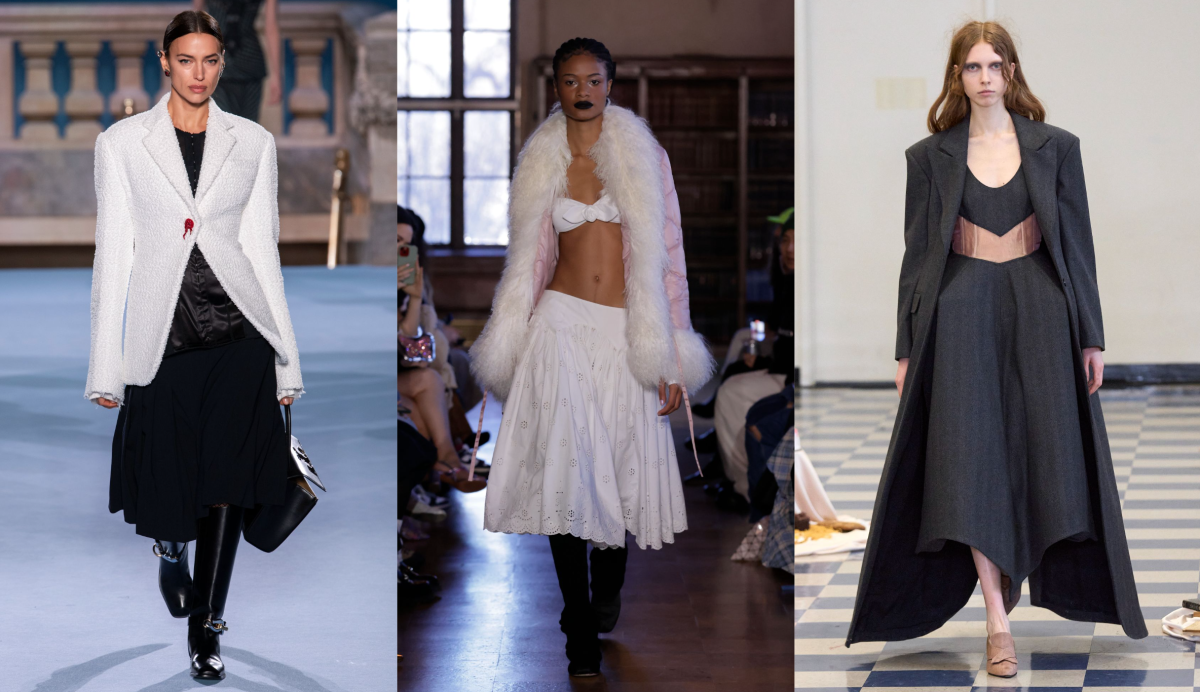The image features a series of three runway models, each showcasing distinctly styled outfits. On the left, a tall, slender model with Mediterranean or Hispanic features is dressed in a striking ensemble. She wears a white fuzzy blazer with oversized cuffs extending to her knuckles, buttoned with a single prominent red button. Underneath, she sports a black satin top paired with a calf-length black skirt, and completes her look with high black leather boots and a black leather purse held in her left hand.

In the center, a model of African heritage with braided or cornrowed hair pulled back displays a vibrant, eclectic outfit. She dazzles in a shiny pink quilted coat with white fur collar and cuffs, which drapes open to reveal a bandeau-style white top adorned with a small central bow. Her midriff is exposed, transitioning into a white skirt with intricate eyelet detailing and a scalloped hem. She complements her look with knee-length black boots, silver glitter eye makeup, blush, and bold black lipstick.

The model on the right, of pale complexion with wavy, reddish-brown hair, brings an avant-garde feel to the runway. She is adorned in a very long black trench coat resembling a blend of a suit jacket and cape. Beneath the coat, she features a black and cream ensemble that forms an angular, downward-pointing design. This consists of a top and skirt that mirror this design and extend into tan loafers or heels, completing her minimalist, grunge-inspired look with nude lips and dark eye shadow.

Together, these models present a compelling visual narrative of contrasting textures, colors, and cultural influences in fashion.